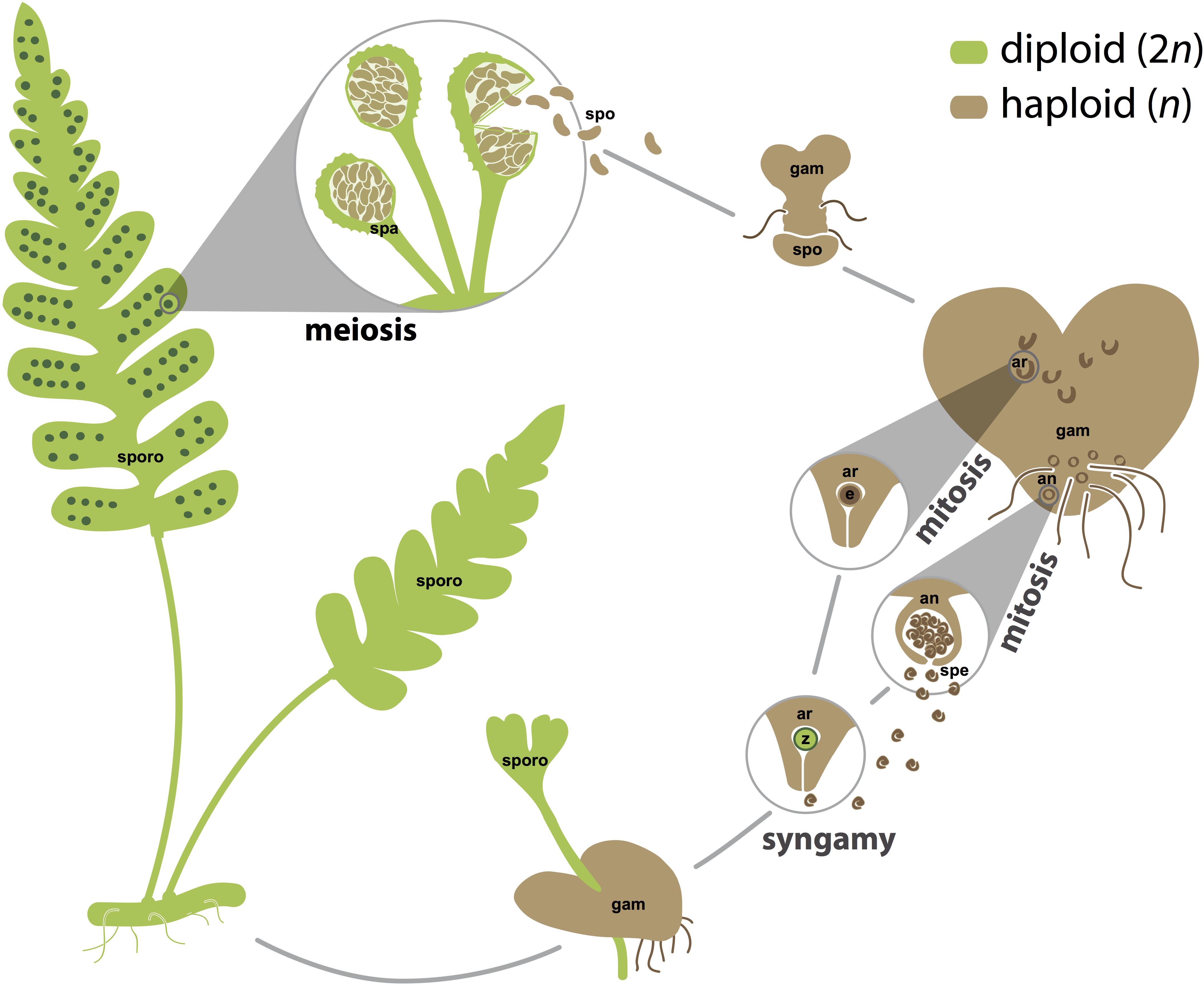This image, set against a white background, appears to be a detailed biological diagram from a scientific journal or textbook, illustrating the life cycle of a plant, likely focusing on the alternation of generations in ferns. The process is depicted in a circular format, emphasizing the recurring nature of the cycle. The diagram is divided into green and brown sections, representing diploid (2n) and haploid (n) stages, respectively. 

On the left side, starting from the bottom, there are green leaves labeled "sporo" symbolizing the sporophyte stage. This is followed by a depiction of spores that undergo meiosis. An arrow points to a small sprout emerging from the soil, labeled "gam," symbolizing the gametophyte stage. As the cycle progresses, the diagram shows processes labeled “syngamy” and several instances of “mitosis.” 

In the upper part, the green area is labeled "diploid (2n)" and the brown area "haploid (n)." The cycle includes detailed images of spores on the ferns and various stages of plant development, with arrows indicating the flow from one stage to another. The document aims to elucidate plant reproduction, alternating between phases of growth and meiosis, illustrated with detailed botanical drawings and scientific notations.